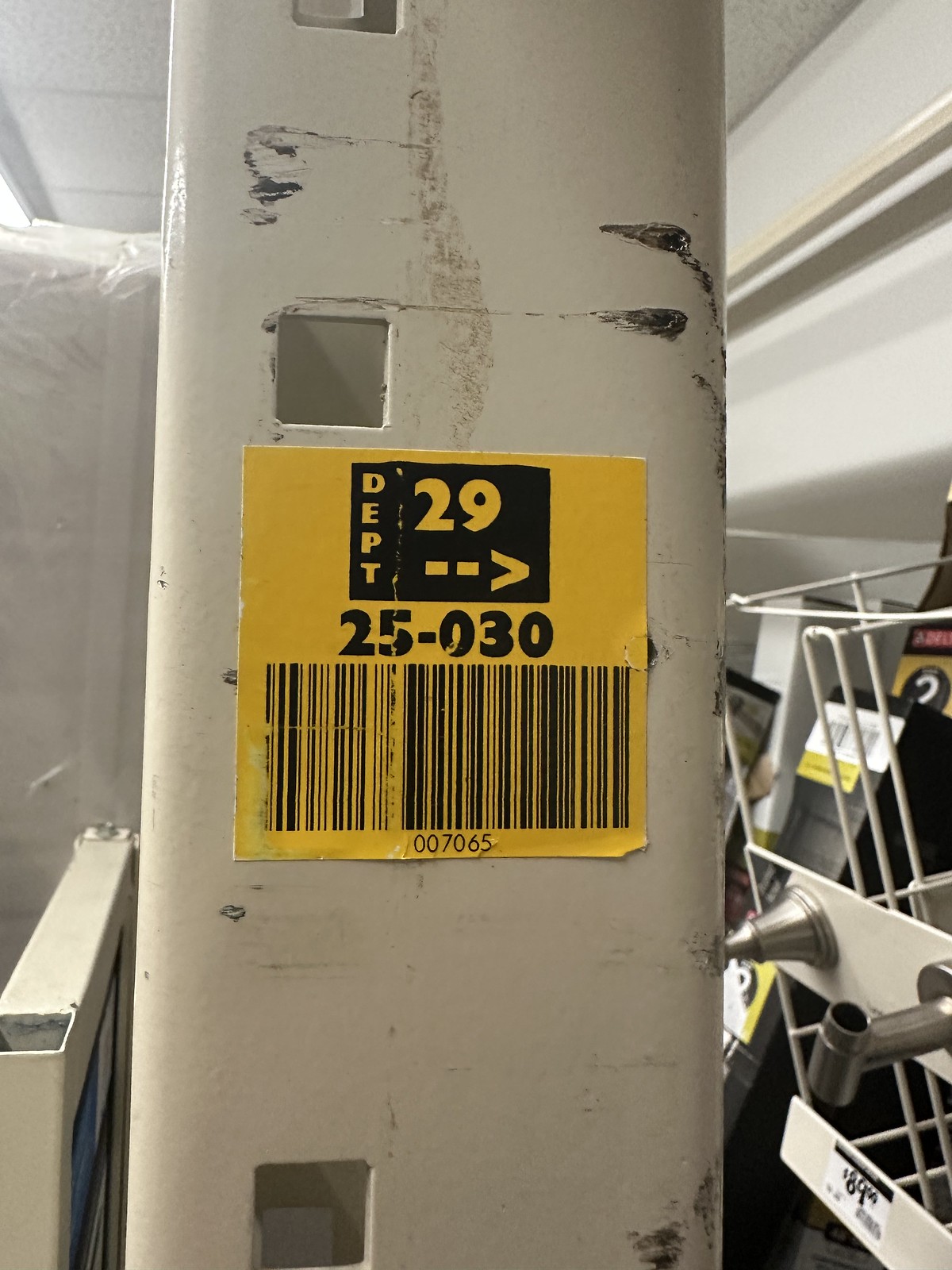A cream-colored beam, marked with numerous black scuff marks, stands prominently in the foreground of a store setting. Shelves lined with various products and price tags fill the background, suggesting a retail environment. Central to the image is a yellow sticker affixed to the beam. The sticker features a barcode and several details: "Department 29" with an arrow pointing to the right, the number "25-030" beneath it, and "007065" under the barcode. The sticker is positioned in the middle of the beam, highlighting its utilitarian function within the store.